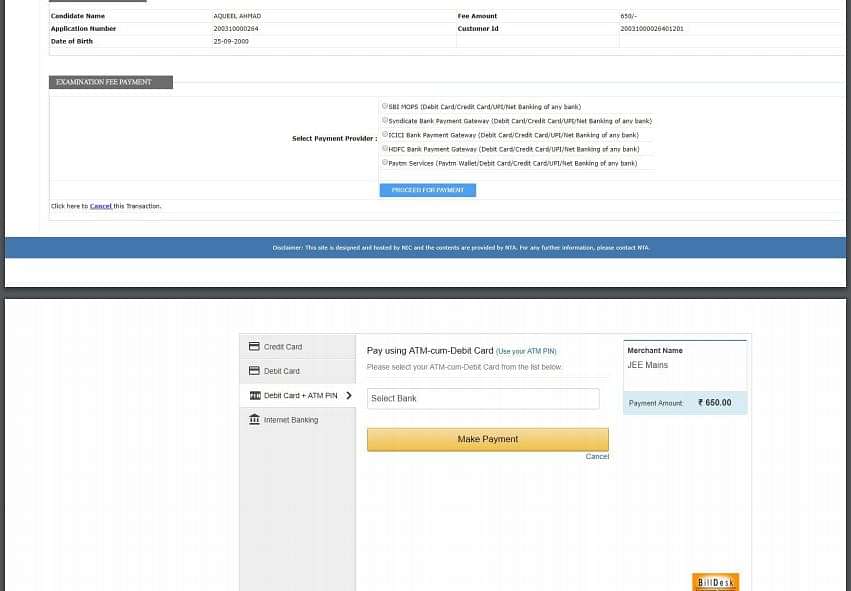**Detailed Caption:**

The image displays what appears to be an online payment page, possibly for an Amazon transaction or a similar platform, identified by familiar button designs. The page is divided into two sections. 

The upper section has a white background and contains a table with three rows of information: 
- The first row labels "Candidate Name," though the name "Akhil Amal" is blurry.
- The second row displays "Application Number" as 200310000264.
- The third row is "Date of Birth," which is partially obscured but lists "25th of September 2000...".

To the right, it mentions the fee amount, $56, immediately followed by a field for "Customer ID" with the same application number appended with 01201.

Below the table, a gray box with white text reads "Examination Fee Payment." Following this is a selection field for payment providers, featuring five options in black text. Below the selection field, a blue button, likely labeled "Process Payment," is positioned.

In the bottom left corner, there is an option labeled "Click here to cancel this transaction," and beneath it, a long blue banner with a white text disclaimer that includes a warning. 

A black bar separates this section from the lower half. The lower section also has a white background and contains a left-side gray menu. The menu lists payment options with avatars:
- "Credit Card" and "Debit Card" Option with a credit card icon.
- "Debit Card and ATM Pin" Option featuring a black box with "PIN."
- "Internet Banking" Option represented by an institutional building icon.

The screen prompts the user to "Pay using ATM..." (the exact text is unclear), directing them to select their ATM debit card from a provided list.

A yellow tab at the bottom of this section encourages the user to "Make Payment."

On the right, the merchant's name "Jemain" (J-E-E-M-A-I-N-S) is displayed, followed by a blue bar indicating the payment amount of $650 in an unspecified currency.

At the bottom right corner of the screen, there's an orange box, which appears to be labeled "Bill Desk" or similar, though it’s difficult to discern clearly.